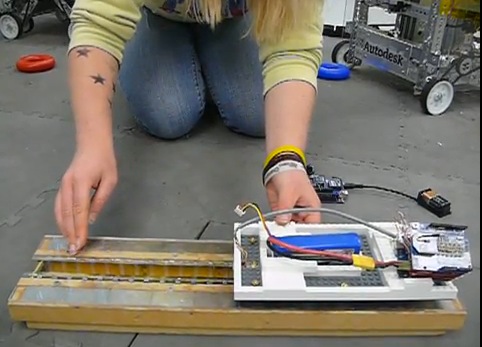In this low-resolution, pixelated image taken from a video, a young girl with blonde hair, dressed in a yellow hoodie pulled up to her elbows and blue jeans, is kneeling on a gray padded floor in a workshop. She is working on an intricate piece of electrical equipment perched on a rustic wooden cradle, surrounded by red and grey electrical cords. Her right forearm displays black star tattoos, while her left wrist is adorned with yellow, black, and white bracelets. A 9-volt battery lies near the equipment. Behind her, there are several metal carts with gears and wheels, possibly motorized carts or robots, one of which has "Autodesk" written on it. The background features red and blue plastic donut-shaped objects scattered on the floor.